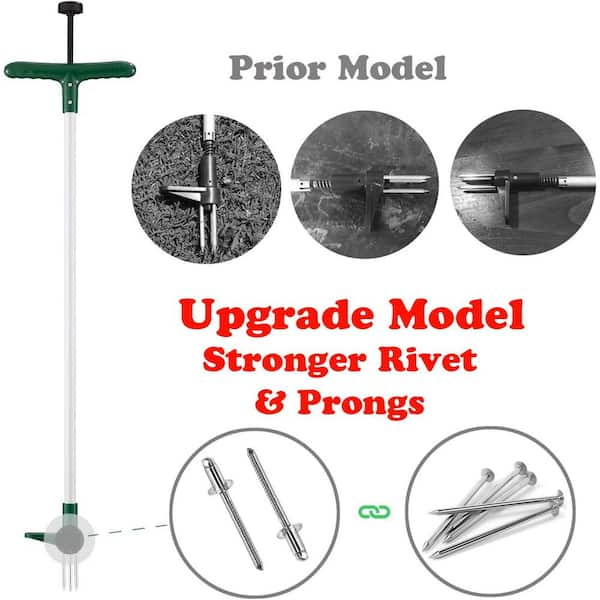The image is an instructional photographic comparison between two models of a tool designed for working with rivets. The background is white, providing a clear canvas for the visual details. The left side of the image features the phrase "prior model" in gray letters, with a close-up of a tool showing a black T-shaped handle attached to a long pole, ending in a gray circular element. Dotted lines lead to a larger section illustrating the old model's rivets.

A green set of chains connects to another rounded element featuring several silver nails, indicating part of the tool's mechanism. The top part of the image highlights "upgrade model" in red, showcasing the improvements. Close-ups of the newer model emphasize a stronger rivet and enhanced prongs. The two models are visually compared, with the older model situated above and the upgraded version below, outlining the physical differences in their mechanisms. The upgraded tool exhibits more robust elements that suggest durability and improved functionality.